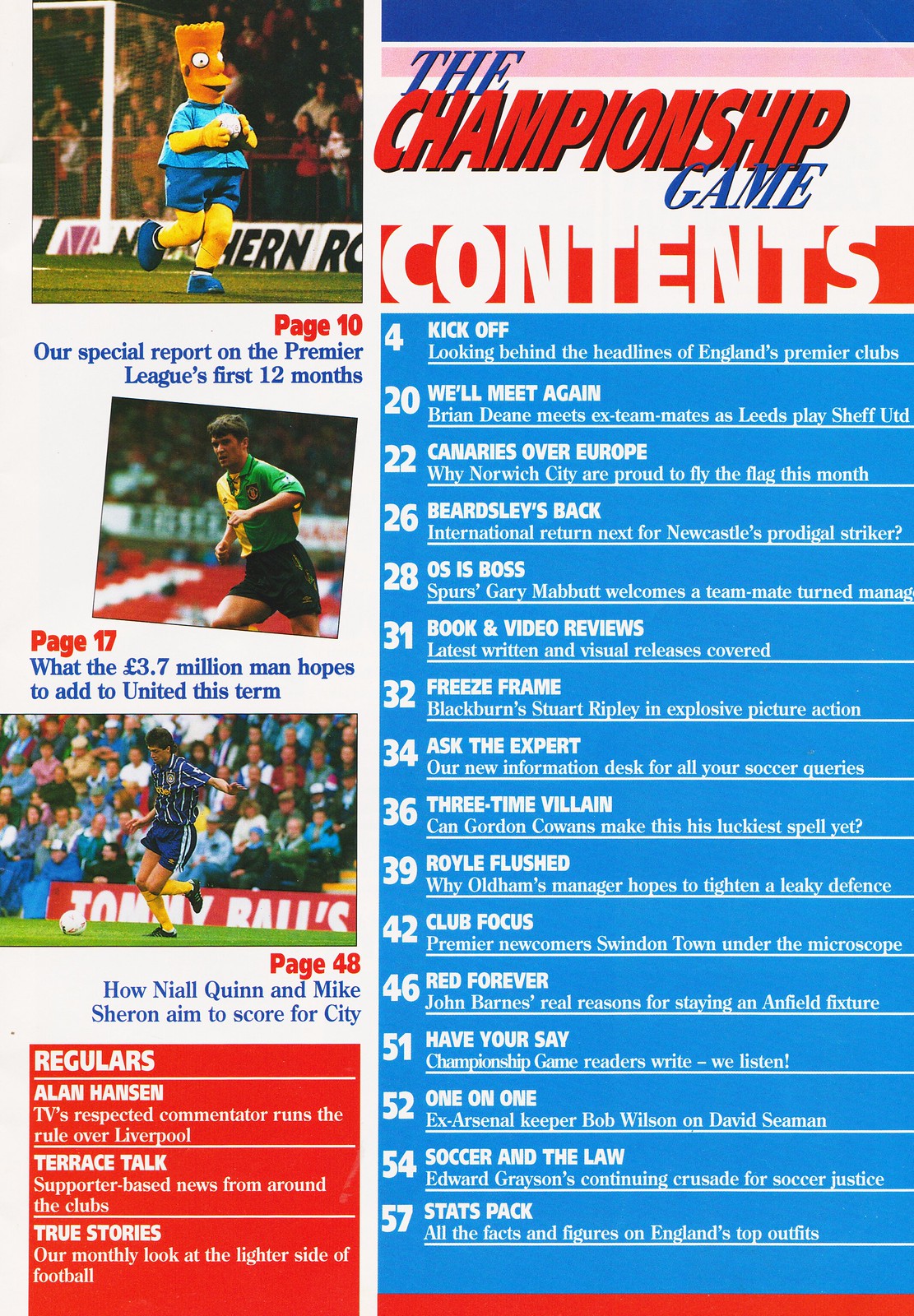This image appears to be a scan of a vintage magazine's table of contents page dedicated to a championship soccer game. Set within a rectangular layout, the left side features a series of evocative images and captions, each highlighting key articles and coverage within the issue. Starting from the top, a colorful shot captures a Bart Simpson mascot in a blue shirt sprinting across a soccer field, holding a soccer ball. This image references a special report on page 10 about the Premier League's first 12 months. Below, a soccer player in a yellow and green kit showcases athletic prowess, with the caption explaining on page 17, the 3.7 million pound man’s ambitions for United. Further down, another action shot presents a player in a blue uniform with white stripes, preparing to kick the ball, which directs readers to page 48's article on Niall Quinn and Mike Sheron's scoring strategies for City. 

To the right, a blue vertical box effectively organizes the magazine's wide range of content, titled "Championship Game Contents," resembling a detailed table of contents. Key sections include:
- Page 4: Kickoff
- Page 20: We'll Meet Again
- Page 22: Canaries Over Europe
- Page 26: Beardsley’s Bag
- Page 28: OS is Boss
- Page 31: Book and Video Reviews
- Page 32: Freeze Frame
- Page 34: Ask the Expert
- Page 36: Three-Time Villain
- Page 39: Royal Flush
- Page 42: Club Focus
- Page 46: Red Forever
- Page 51: Have Your Say
- Page 52: One on One
- Page 54: Soccer and the Law
- Page 57: Stat Pack

Further insight reveals the "Regulars" section in a distinct red box, featuring segments like "Regulars," "Alan Hansen," "Terrorist Talk," and "True Stories", which offers a blend of commentary, fan engagement, and light-hearted features. This amalgamation of captivating visuals and thorough content breakdown provides readers an enticing preview of the magazine’s comprehensive soccer coverage.